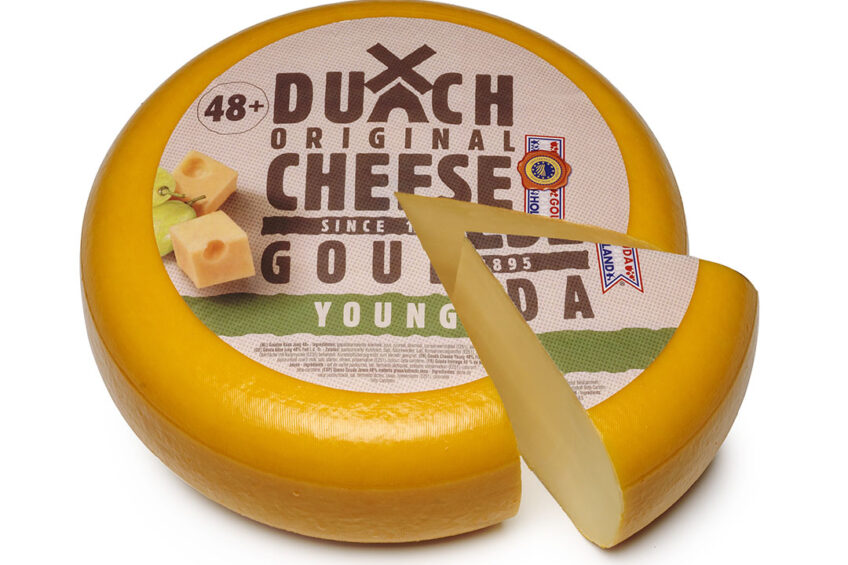This image depicts a round wheel of cheese with a small wedge removed at approximately the five o'clock position. The cheese, likely Gouda, appears to have a waxy outer coating and features a detailed label on its top. The label reads "Dutch Original Cheese since 1895" with the word "Dutch" styled such that the "T" is represented by a windmill. Below this, the label specifies "Gouda Young" in white text on a green strip, and to the left is a circular emblem with "48 Plus." The text is primarily in brown font. Additionally, the label shows an illustration of two cheese cubes and some grapes, suggesting possible pairings. There is a vertical label on the right side of the wheel, which includes "Gouda" and "Holland." The wedge that has been cut out appears to be slightly pulled away from the main wheel.